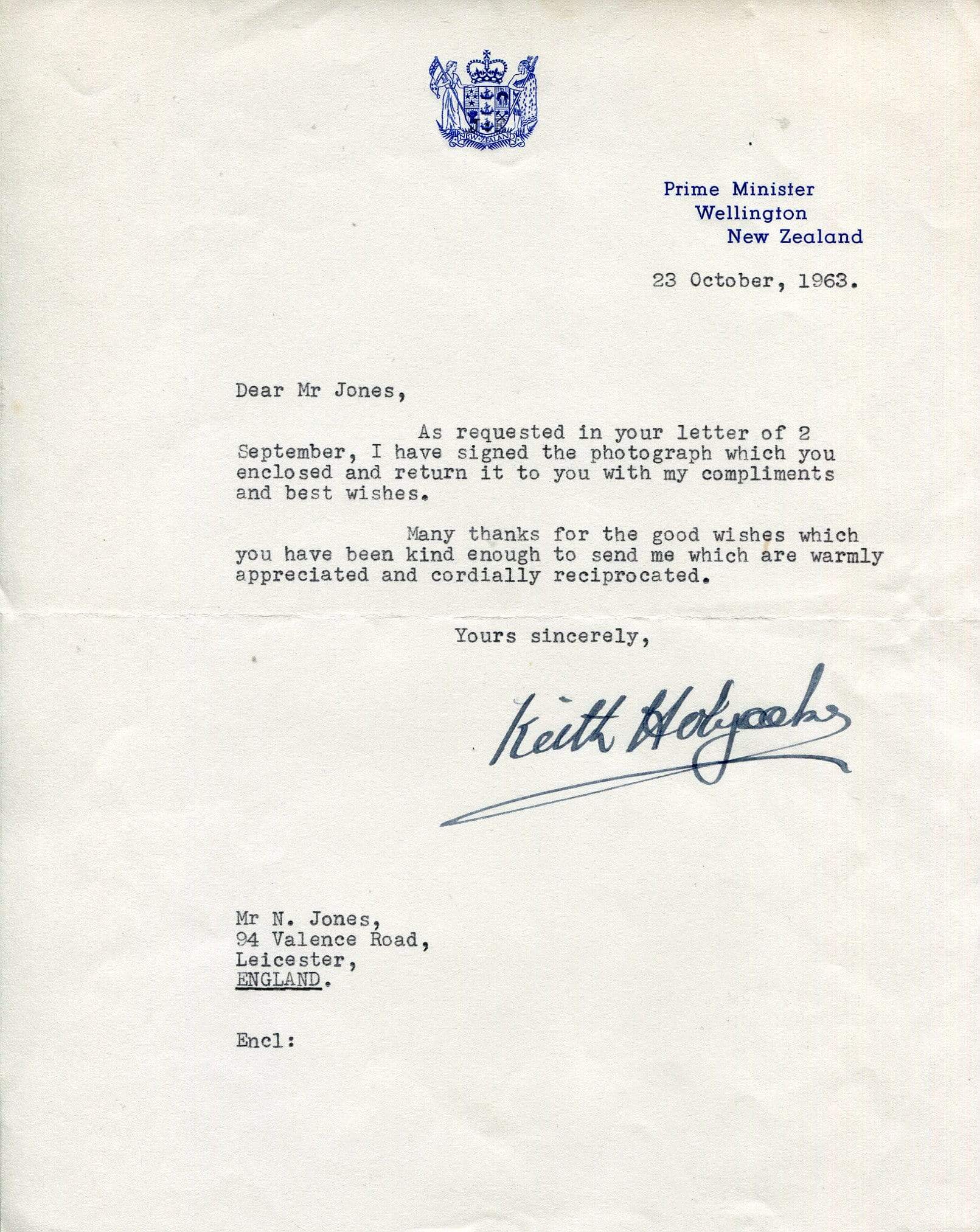The image depicts an old letter photographed in detail. The letter, dated 23rd October 1963, is typed on white paper of standard letterhead size, showing signs of age with a crease running horizontally across the center. At the top center, there is a blue crest featuring two figures flanking a central shield and sword motif crowned at the top. The top right corner of the letterhead reads "Prime Minister Wellington, New Zealand." 

The content of the letter is as follows:
"Dear Mr. Jones, 
As requested in your letter of 2 September, I have signed the photograph which you enclosed and return it to you with my compliments and best wishes. Many thanks for the good wishes which you have been kind enough to send me, which are warmly appreciated and cordially reciprocated. 
Yours sincerely, 
[signed in blue ink] Keith Holyoake."

The rest of the text is typed in black, while the signature after "Yours sincerely" is notably in blue ink. The address, "Mr. N. Jones, 94 Valence Road, Leicester, England," is typed at the bottom left of the letter. The letter encloses a signed photograph as per Mr. Jones's request.